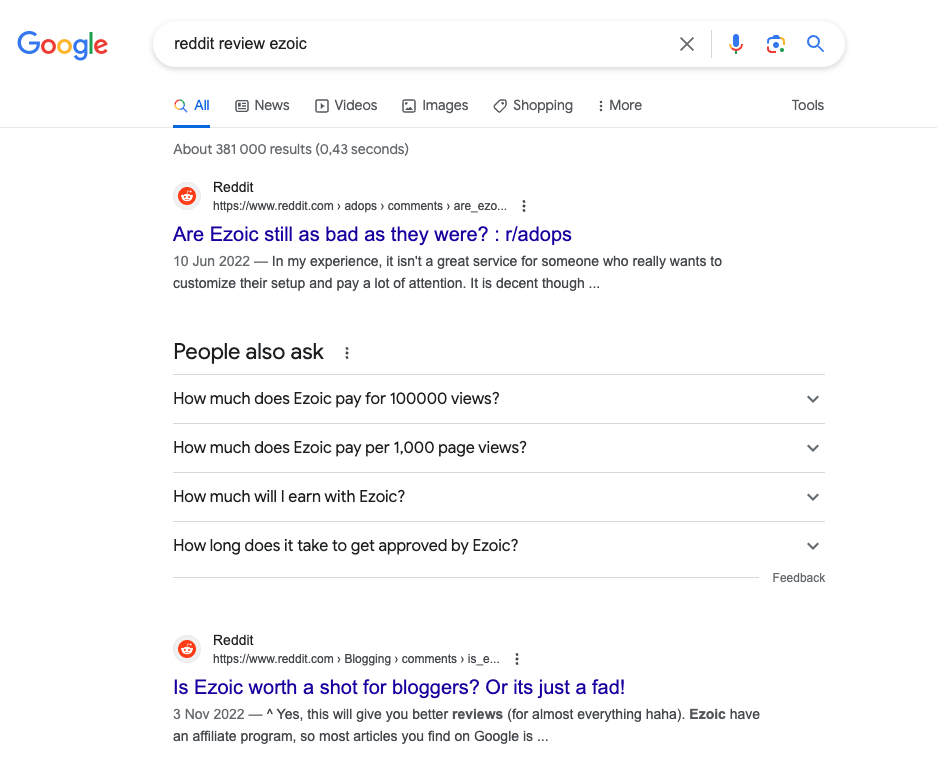The image depicts a Google search results page for the query "Reddit review E-Z-O-I-C." At the top, the familiar Google search box displays this query. Below the search box, standard navigation tabs are visible, including "All," "News," "Videos," "Images," "Shopping," "More," and "Tools." The page reports approximately 381,000 results found in 0.43 seconds.

The first result features the Reddit icon and web address. The linked text in blue reads, "E-Z-O-I-C still as bad as they were? : r/adops." The posted date is June 10th, 2022. An excerpt follows: "In my experience, it isn't a great service for someone who really wants to customize their setup and pay a lot of attention. It is decent though."

Scrolling further, a "People also ask" section appears, presenting commonly searched questions related to E-Z-O-I-C: 
1. "How much does E-Z-O-I-C pay for 100,000 views?"
2. "How much does E-Z-O-I-C pay for 1000 page views?"
3. "How much will I earn with E-Z-O-I-C?"
4. "How long does it take to get approved by E-Z-O-I-C?"

The second search result again features the Reddit icon and web address. The linked text in blue reads, "Is E-Z-O-I-C worth a shot for bloggers or just a fad!" with a posting date of November 3rd, 2022. The excerpt provided mentions, "Yes, this will give you better reviews for almost everything. Ha ha. E-Z-O-I-C have an affiliate program. So most articles you find on Google is."

The screenshot provides an insightful summary of user opinions and common inquiries about E-Z-O-I-C, as seen on Reddit and compiled by Google's search algorithm.